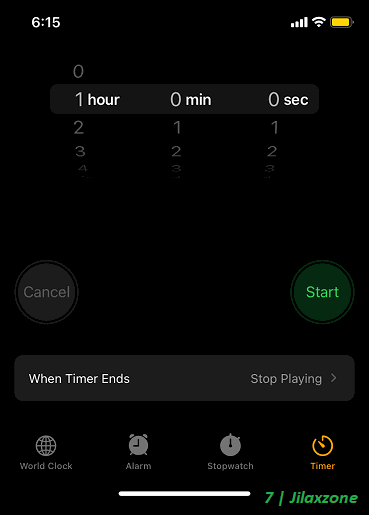In this image, the top right corner displays a yellow battery icon turned on its side. Next to it, towards the left, is the Wi-Fi signal strength icon showing full bars, followed by the phone signal strength icon, also at full bars. The current time, located at the top left, reads 6:15.

Below the time, a timer interface is visible. The far left section represents hour markers labeled 0, 1, 2, 3, and 4, with the number 1 currently selected. In the middle section, the minute timer is displayed, marked 0, 1, 2, and 3, with the number 0 selected. The rightmost section displays the second timer, also numbered 0, 1, 2, and 3, with the number 0 highlighted.

In the central part of the image, slightly toward the bottom left, there is a dark gray circular button labeled "Cancel." Towards the bottom right is a green button labeled "Start," with the word "Start" in a lighter shade of green.

Below this, within a boxed area, there is a setting labeled "When Timer Ends" on the left side and "Stop Playing" on the right. Finally, at the very bottom center of the image, four icons are visible: World Clock, Alarm, Stopwatch, and Timer.